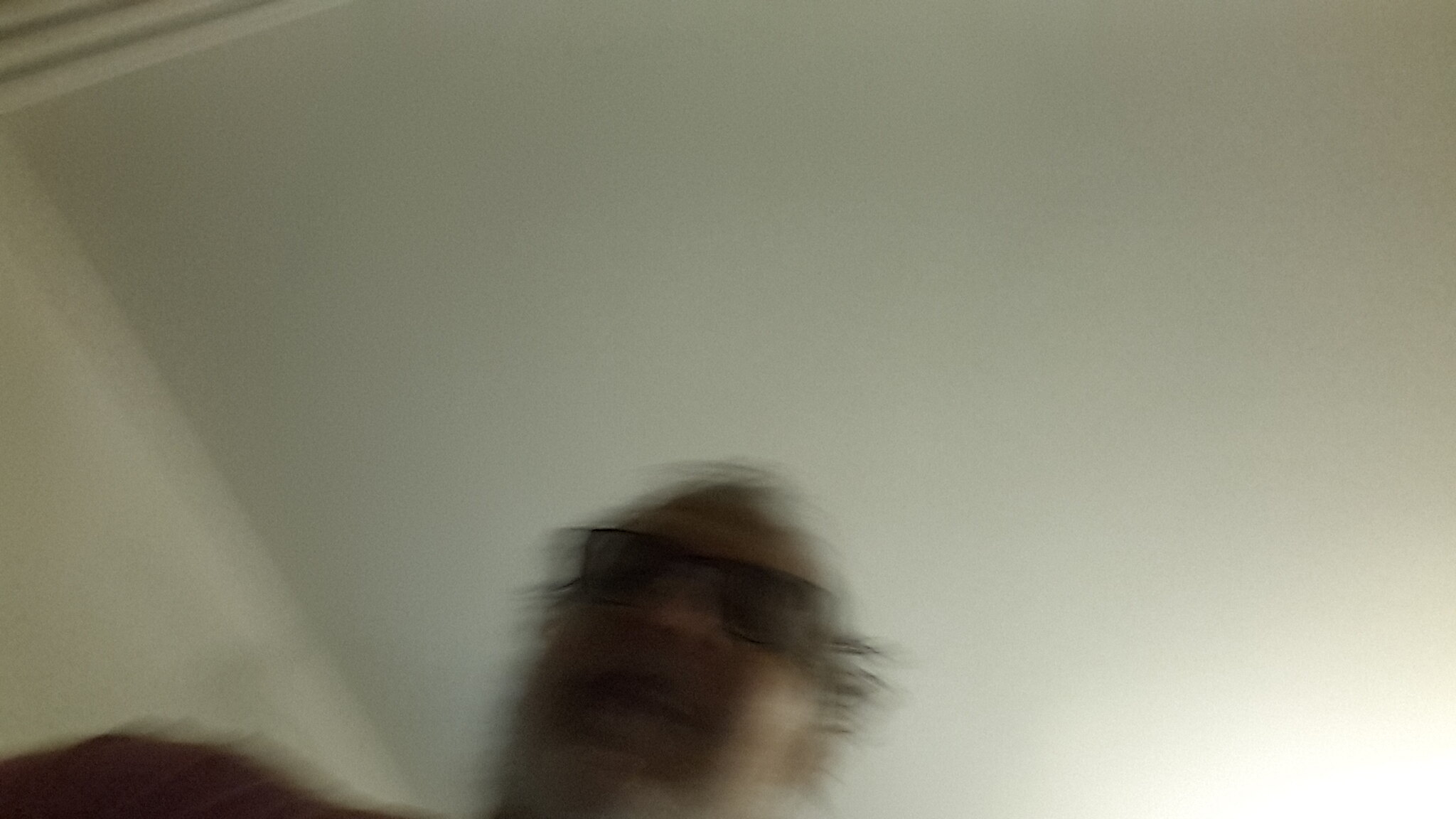The photograph captures a slightly jagged and blurry image of an older man, possibly in his 50s or 60s, looking down into the camera, suggesting the shot was taken from a low angle. His head and part of his shoulder, clad in a dark red shirt, dominate the composition. The man sports white and gray hair, a goatee, and sunglasses which obscure his eyes. The background reveals a white or cream-colored ceiling with molding, indicating the setting is an indoor white room. There is a bright light source just outside the frame on the right, causing a noticeable glare in the image. Despite the blur, the man seems to be smiling slightly.